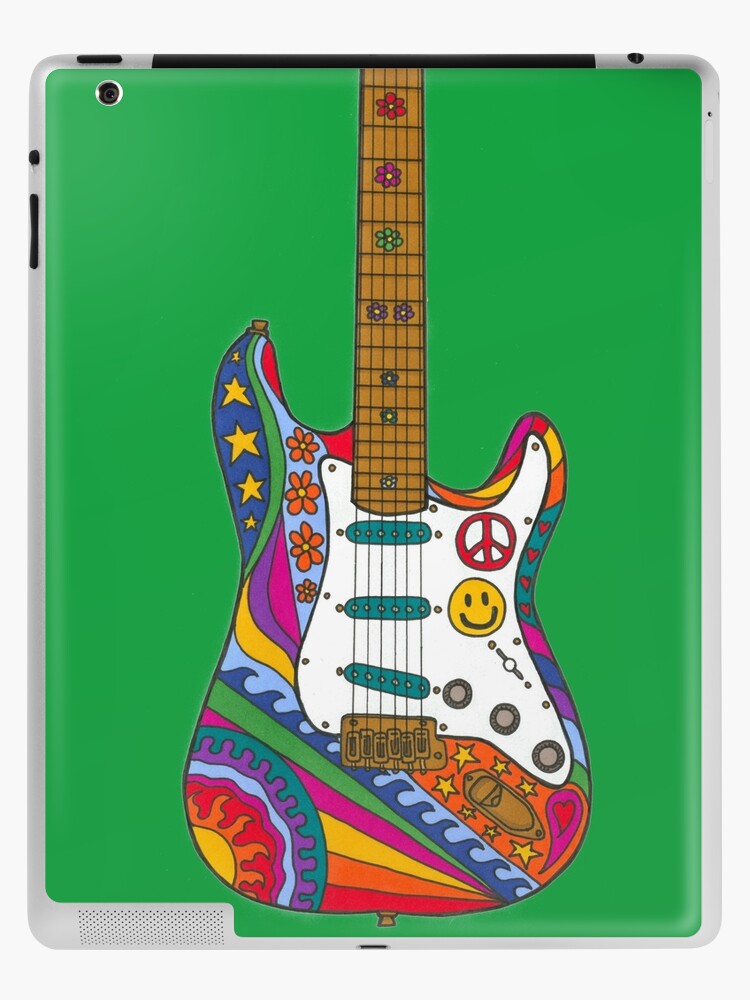The image depicts a brightly colored, psychedelic-themed iPad cover with a vibrant green background. At the center of the cover is a stylized electric guitar adorned with intricate, hippie-inspired graphics. The guitar features a kaleidoscope of colors, including rainbow hues, and is embellished with various whimsical elements. Yellow, orange, red, purple, teal, and blue stripes blend seamlessly with hearts, flowers, stars, and sunshine. Near the strings on the left side are iconic symbols such as a peace sign and a smiley face, while additional flower designs embellish the neck and fretboard of the guitar. The iPad itself sits on a clean white background, highlighting the vivid contrasts and details of the psychedelic artwork.